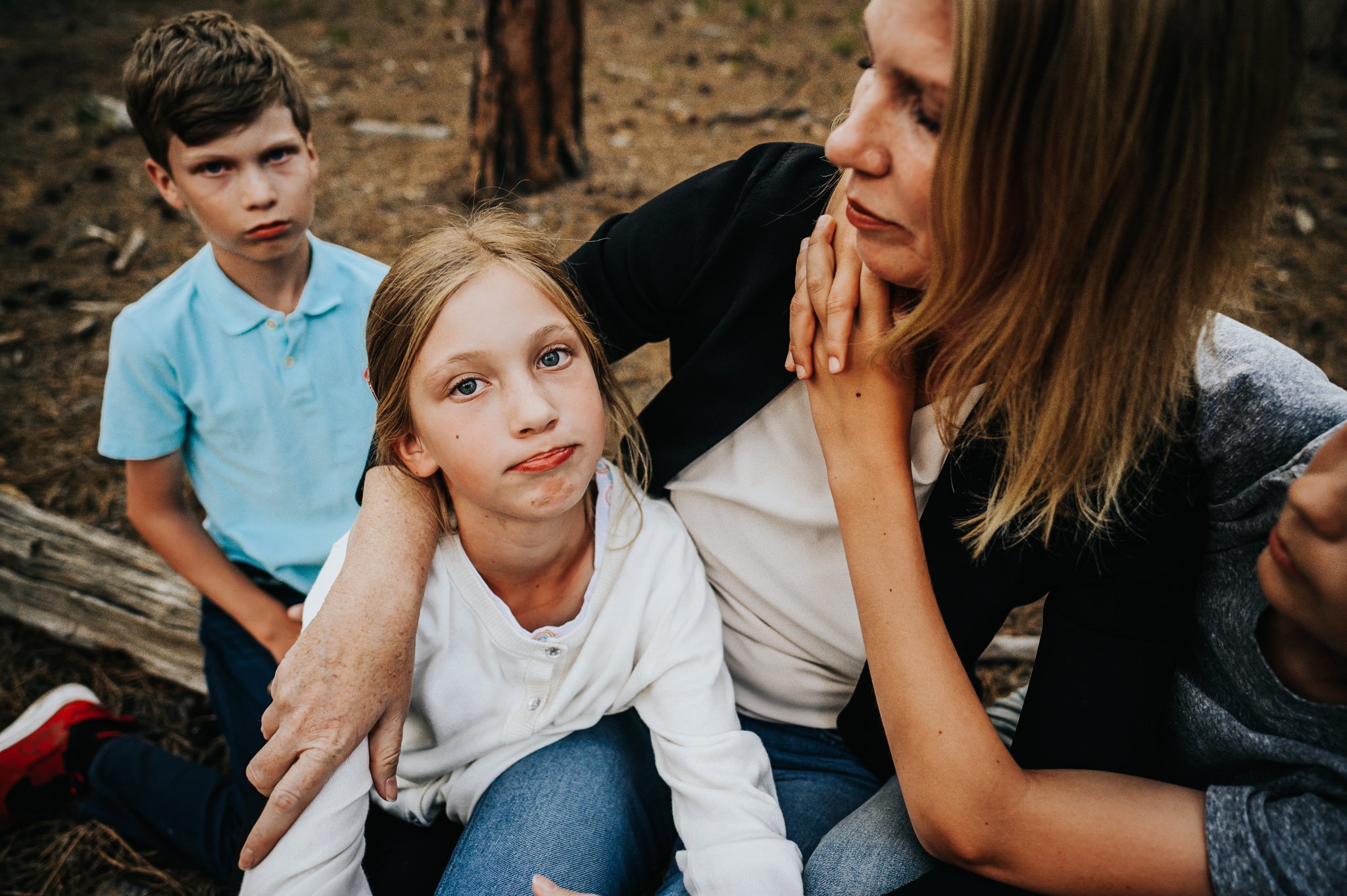The image portrays a family of four, likely a mother and her three children, captured in a slightly somber and candid moment outdoors. The mother, centered in the image, has longer brownish hair and is dressed in a black sweater over a white t-shirt, paired with blue jeans. To her immediate left, her arms encircled by the mother, is a young girl of around seven or eight years with brownish-blonde hair and blue eyes, wearing a white top and blue jeans. The girl is noticeably not smiling. On the mother's right side, partly cut off from view, is a young boy in a gray shirt hugging her, his face obscured as his arms are wrapped around her neck. Standing to the far left, close to the mother, is another boy, who appears slightly younger than the girl. He has brown hair, a light blue polo shirt, and is looking stoically at the camera, also not smiling. The setting appears to be outdoors near a tree, although the focus remains closely on the family members, highlighting their expressions and attire in what looks like a casual, yet reflective moment.